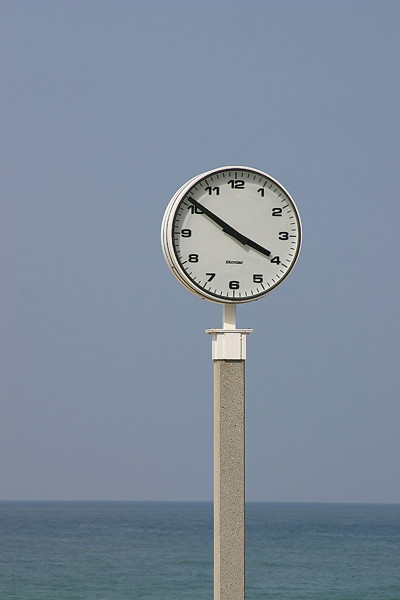A striking outdoor photograph features a white, circular clock prominently positioned in the center of the image. The background showcases a stunning body of turquoise to dark blue water that gradually meets a serene blue sky at the horizon. The clock, attached to a tan, rectangular, concrete pole with a white cap, appears to be emerging from the water. It has a bold black border and black numbers from one to twelve with two black hands indicating the time as 3:51. The rectangular base of the clock secures it firmly to the pole, lending a unique and somewhat surreal impression, as though the clock is floating on the water's surface.